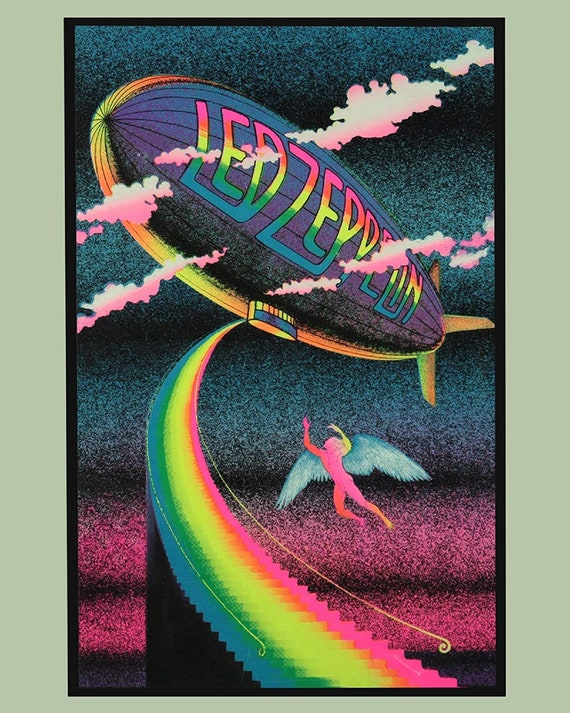The image is an artistic depiction framed with a black border against a light green-gray wall, resembling a promotional poster for Led Zeppelin. Dominating the composition is a colossal blimp, painted with shades of purplish pink and vibrant hues of yellows and greens. The side of the blimp features the text "Led Zeppelin" in a rainbow-colored palette including purples, pinks, yellows, blues, and greens. The blimp has a lower observation deck, a viewer's box with windows where passengers would stay, and is detailed with fins near its tail, evoking the appearance of a whale. 

Surrounding the blimp are pink-tinted clouds, some of which obscure parts of the Led Zeppelin text. The background exudes a nighttime sky ambience, transitioning from dark blue to light blue hues. At the forefront, a rainbow staircase extends upward from the bottom, curving toward the blimp adorned with light yellow railings. An angelic figure, with a nude, rainbow-colored body and striking white wings, reaches up towards the blimp from the staircase. The lower part of the image portrays a swirling cascade of purplish-pink waves, providing a striking contrast to the overall dark, star-speckled sky.